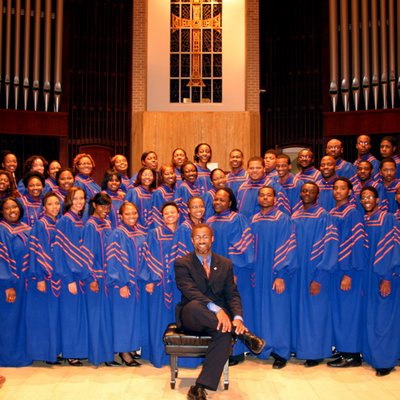The image captures a vibrant, predominantly African American church choir dressed in blue robes accented with gold outlines. The choir is arranged in three ascending rows, suggesting a diverse congregation of younger individuals. Seated prominently at the front is a man who appears to be the preacher or choir leader. He is attired in a black suit, a blue shirt, and a red tie, with his legs crossed comfortably on a padded stool. This man has short black hair, glasses, and black shoes. Behind the choir, a gold cross is mounted on the wall, centered between what seem to be organ pipes. The background and floor feature various wood tones, adding a warm ambiance to the setting. The overall scene exudes a sense of unity and joy, as visible in the smiling faces of the choir members and the preacher.